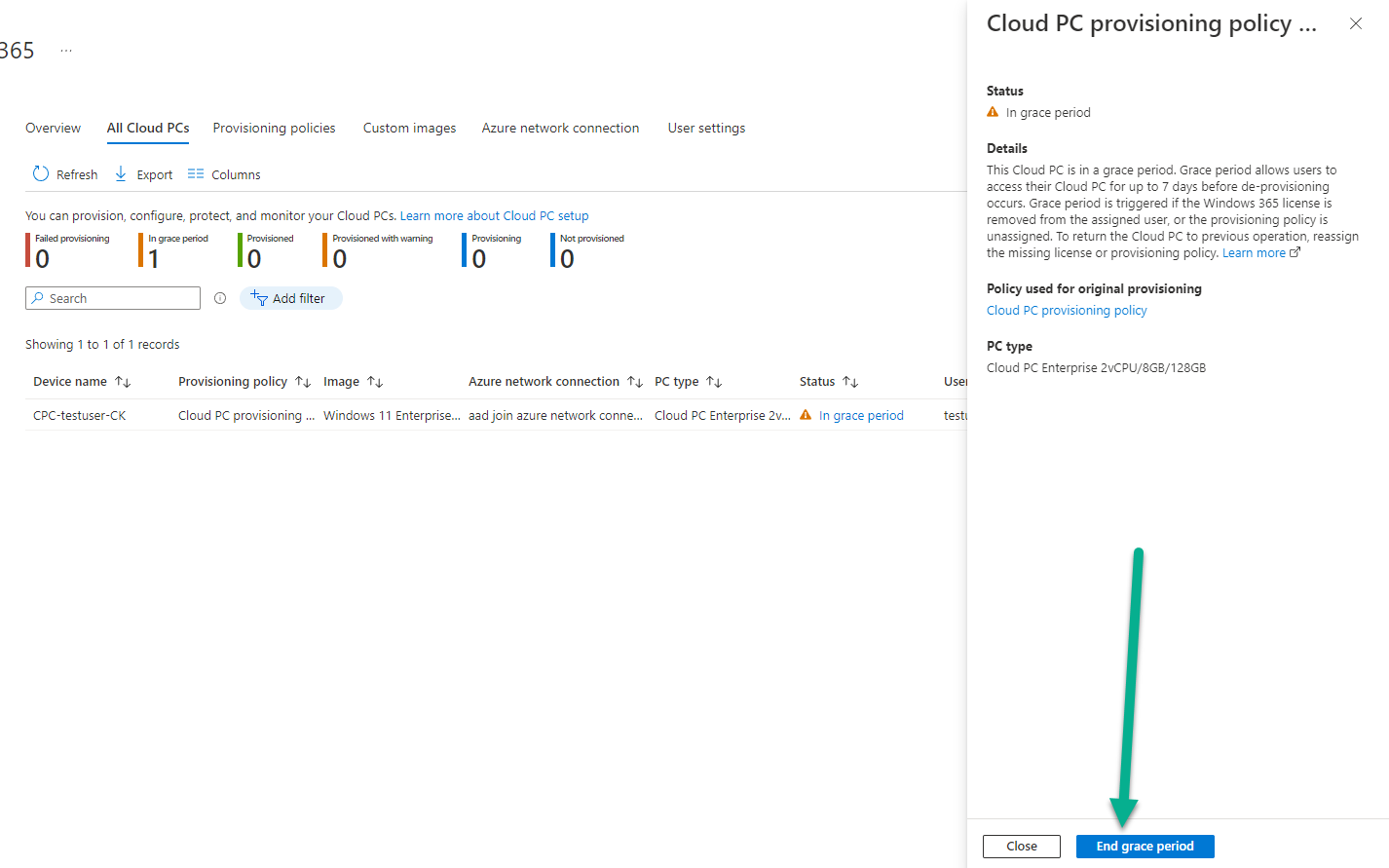**Detailed Caption for Image on Cloud PC Provisioning Policies:**

The image provides a comprehensive overview of cloud PC provisioning policies, focusing on different elements involved in the provisioning process. The highlighted section at the top mentions "All Cloud PCs," and nearby, in the upper left-hand corner, a number is displayed which appears to be either 365 or 865. 

The image enumerates various components such as provisioning policies, custom images, Azure network connections, and user settings. The device name listed includes details like provisioning policies, CPC test user, CK, cloud PC provisioning, Windows Enterprise, AAD joint Azure network connection, and cloud PC Enterprise.

A notable feature in the image is an orange triangle symbol signaling that the status is "In Grace Period." An accompanying detailed explanation informs that this cloud PC is currently in its grace period. This grace period permits users to access their cloud PC for up to seven days before deprovisioning takes place. The grace period is activated if the Windows 365 license is rescinded from the assigned user or if the provisioning policy is unassigned. To revert the cloud PC back to its previous operational status, one must reassign the missing license or provisioning policy.

Highlighted in blue text, there are prompts for users to "Learn More," along with a crucial note that the policy used for the original provisioning is "Cloud PC Provisioning Policy." The PC type is specified as Cloud PC Enterprise, featuring 2V CPU, 8GB RAM, and 128GB storage.

An additional green arrow points downward, indicating options to either "Close" or to "End Grace Period," providing a clear directive for concluding the grace period.